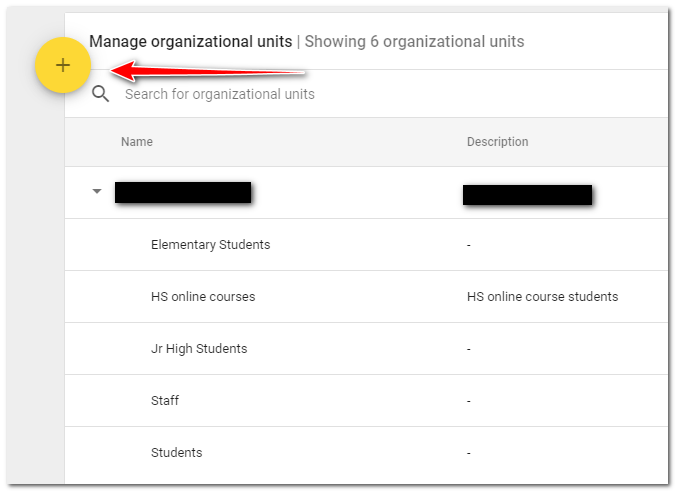The image is a partial screenshot of a web page, possibly displaying a software demo interface. The background is white, creating a clean and minimalistic look. At the very top in dark gray font, the text reads "Manage Organizational Units," followed by "Showing six organizational units" in lighter gray font.

To the left of this text, there is a yellow circle with a black plus sign in the middle, indicating an option for adding elements. A red arrow is pointing to this circle, and beneath the arrow, it reads "Search for organizational units." Directly to the left of this annotation is a small gray search icon, depicted as a magnifying glass (a circle with a line extending to the lower right).

Below this section, there is a light gray rectangle featuring text headers in slightly darker gray font. On the left, the header says "Name," and on the right, it says "Description." Under these headers, black rectangles obscure certain content, suggesting possible content redaction or placeholders.

Underneath these rectangles, the text continues in gray font, listing the organizational units. The "Name" column includes entries like "Elementary Students," "HS Online Courses," "Junior High Students," "Staff," and "Students." Correspondingly, under the "Description" column, the entry "HS Online Courses" is repeated as "HS Online Students." The rest of the lines lack descriptions, offering only unit names.